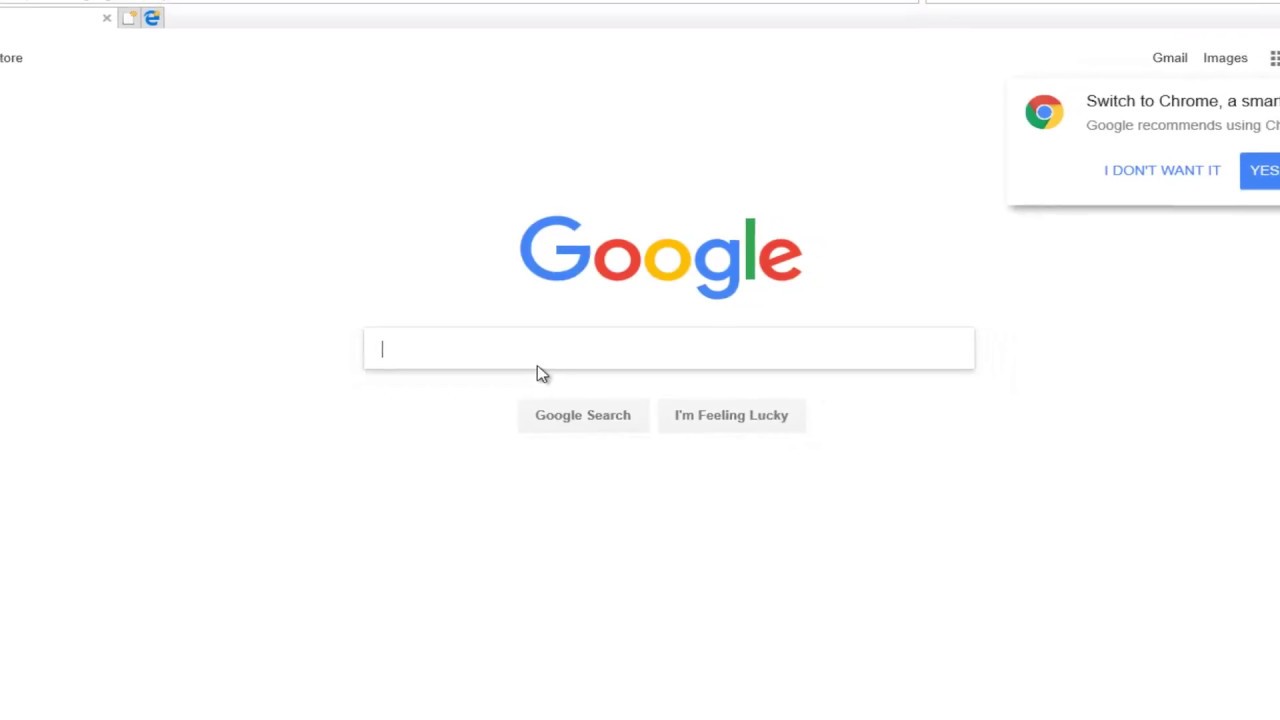On a white background, there's an image depicting a digital interface. In the center, a white square, resembling a piece of paper, prominently displays a capital "E." The top portion features a grid of Gmail icons arranged in three rows of three squares, although the grid is partially cut off. The interface suggests switching to Google Chrome, with the partially visible prompt "Google recommends using Chrome," where only part of the sentence is clear.

Below this, there's a blue button labeled "I don't want it," next to which is a blue square with the word "Yes" in white text. The iconic Google logo appears in its distinctive colors: a blue "G," a red "O," a yellow "O," a blue "G," a green "L," and a red "E." 

A search bar is situated underneath the logo, with a cursor positioned within it alongside a pointer, indicating user interaction. Below the search bar, there are two gray buttons with black text. The first button reads "Google Search," and the second one reads "I'm Feeling Lucky."